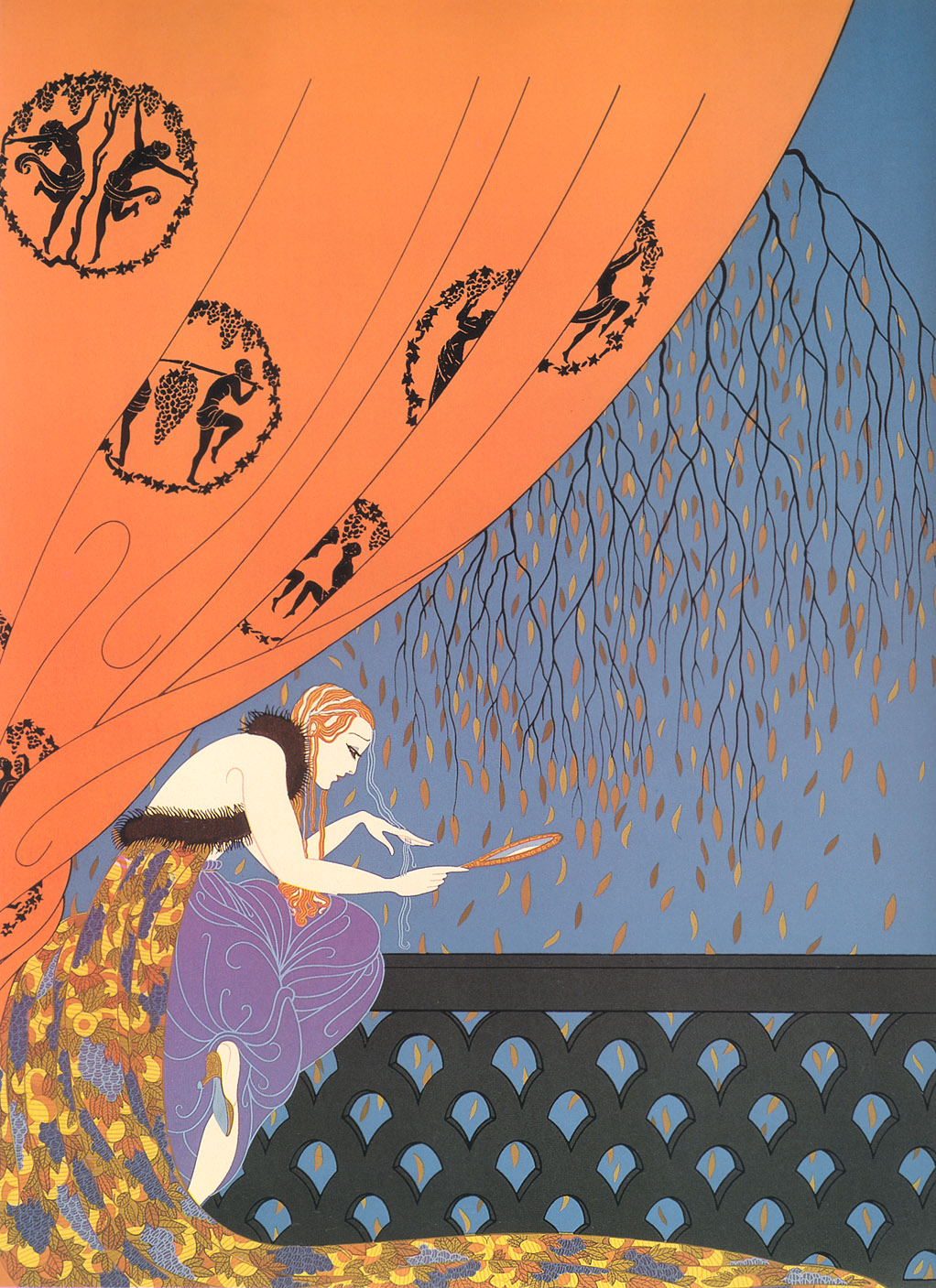In this vibrant and abstract art piece, we see a woman with fair skin and flowing orange hair standing on a deck. She is wearing a striking dress that transitions between shades of purple, yellow, orange, and brown, accompanied by a brown scarf and an eye-catching orange feather. 

Positioned in the bottom left corner of the image, the woman's dress flows gracefully to the right, where it forms what appears to be a long, multicolored tail wrapping around the floor, predominantly displaying hues of purples, reds, oranges, and yellows. She leans on a black, perhaps gray railing with one knee, gazing downward while holding a small mirror. 

Dominating the upper portion of the image are a set of long, dramatic orange curtains adorned with black logos, behind which a tree branch with black limbs and autumnal leaves in shades of yellow, orange, and brown extends into view. The background features elements that resemble a buoyant balloon or orb with intricate hieroglyphics, contributing a sense of whimsy and movement with its orange and blue hues. This captivating image blends surreal and naturalistic elements, making for a compelling and visually striking composition.